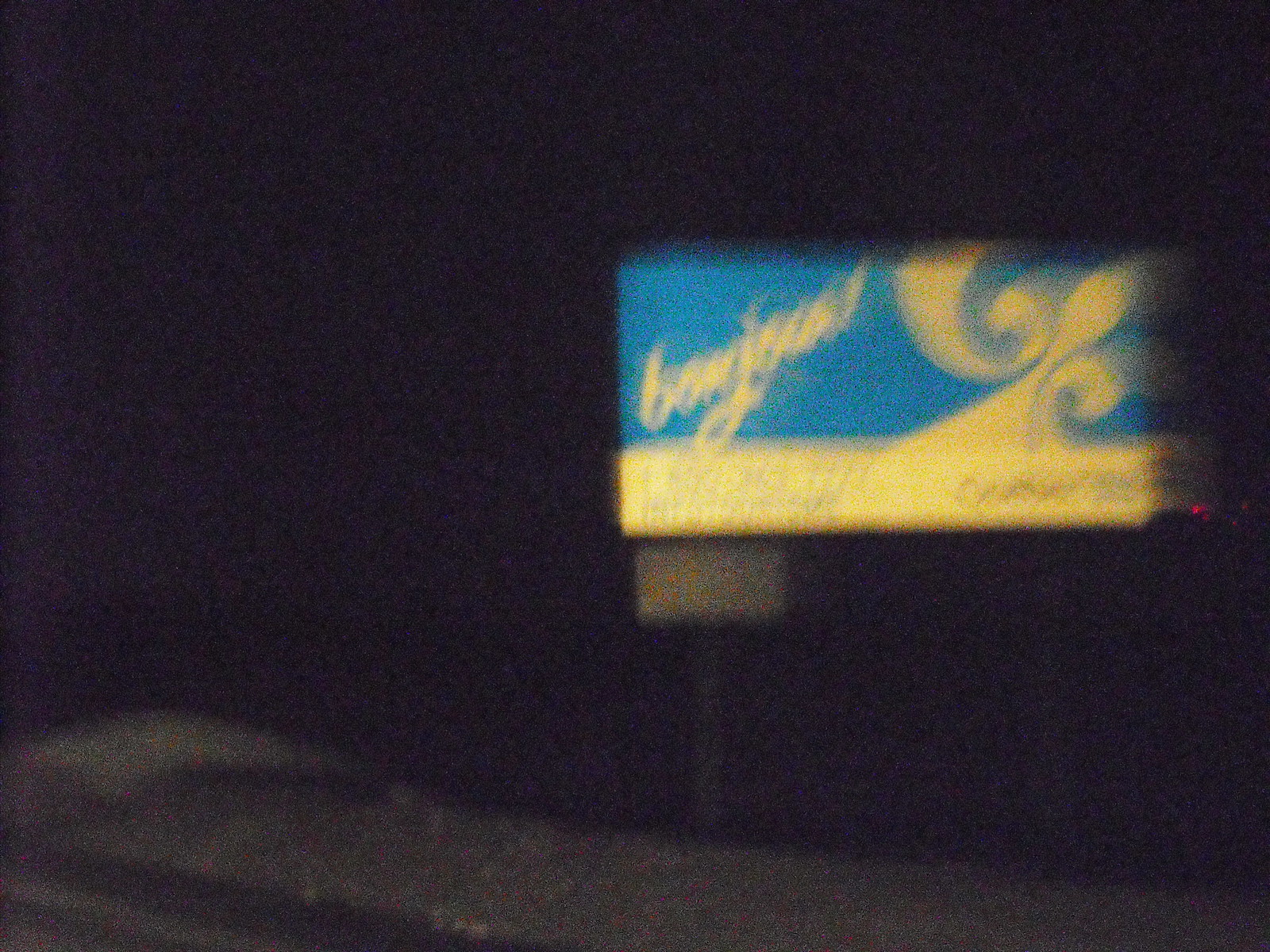This is a color photograph, predominantly dark with an almost entirely black background reminiscent of a night sky. The faint shadows at the bottom are difficult to make out and appear in lighter gray. Towards the center-right, there is a rectangular sign that is very blurry and appears low resolution. The sign features a blue background at the top and a yellow background at the bottom, with the yellow rising on the right in a wave-like design, while the blue has a curved wave coming in from the top and bottom. The top left corner of the sign has diagonal text that seems to spell "bonjour" in cursive, although the blurriness obscures it. There are also some small, indistinct black texts at the bottom right of the sign. Additionally, there is a tiny red light at the bottom edge of the sign. Underneath and slightly to the left of this sign is a smaller, lighter gray rectangle, appearing almost like a paper wrapper. Below this are what seem to be two faint legs. The overall image remains very dark and indistinct.